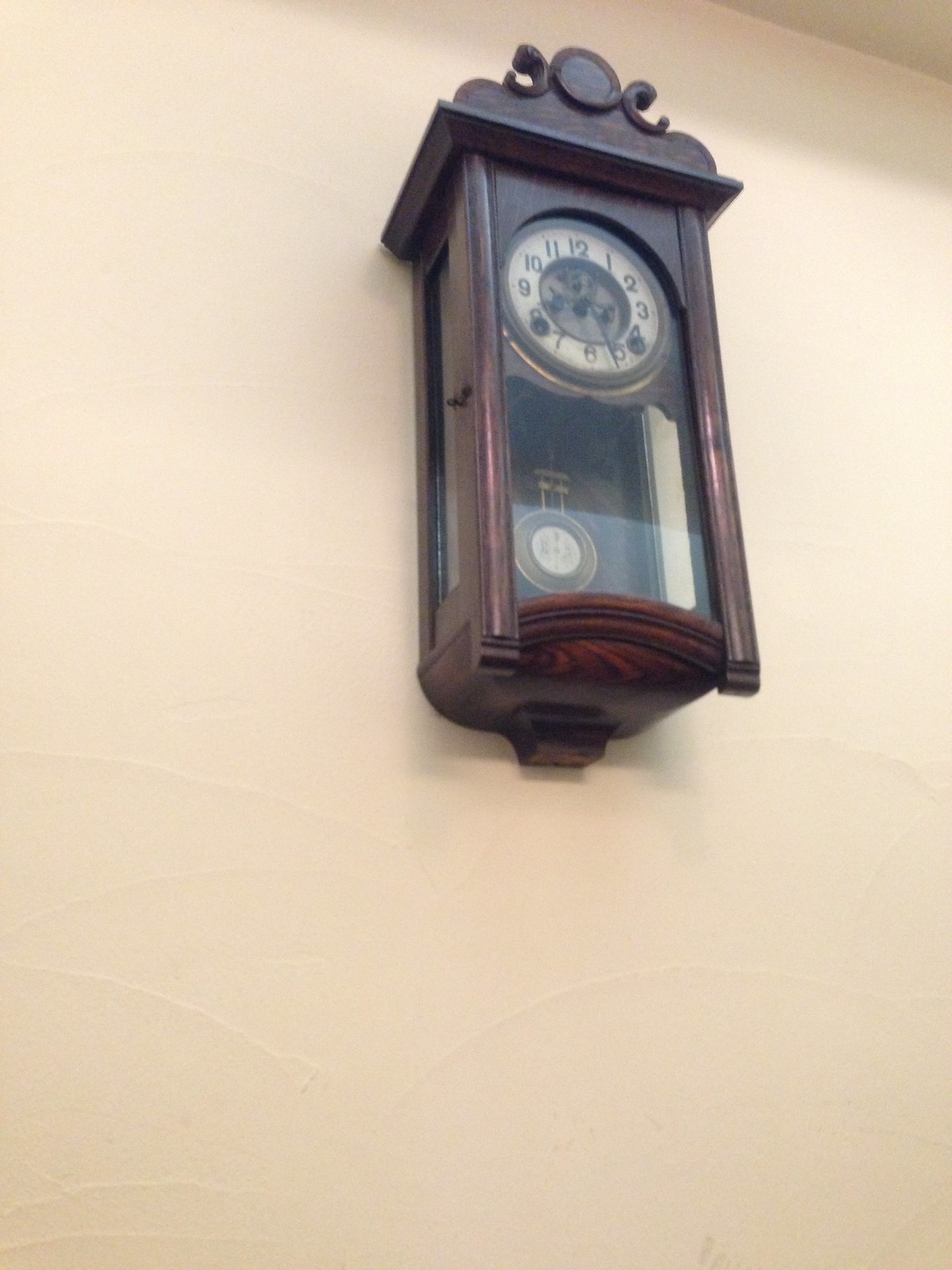This color photograph captures a vintage pendulum clock mounted on a white, textured wall. The clock is encased in rich brown wood and features a glass cover over both the dial and pendulum areas. A latch for the door, located on the left side, adds to its antique charm. The clock's dial is a crisp white, complemented by black hands and numerals. Beneath the clock face, a pendulum with bronze and gold hues dangles elegantly. Atop the clock cabinet, intricate carved scrollwork culminates in a central circular motif, showcasing masterful craftsmanship. Positioned in the upper right quadrant of the photo, the clock stands in sharp contrast to the rest of the image, which is dominated by the plain white wall. The photograph is pristine, devoid of any text, allowing the clock to be the focal point.